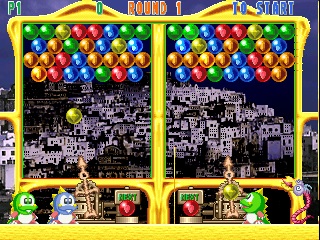The image is a small screenshot from an old video game reminiscent of those found on a color Game Boy, with low-resolution graphics. The game screen features a yellow base or flooring across the bottom, with two small caricature dinosaurs on the left and one on the right. These dinosaurs have spines comprised of yellow triangles extending from the top of their heads down to their tails and slightly open mouths revealing two white, outward-facing buck teeth. 

At the top of the screen, "Round 1" is displayed in orange text centered, and "P1" in green is shown on the top left. To the top right, blue text reads "To Start" along with two blue stars. The top part of the game screen is predominantly blue, transitioning to a background of bunched-together, white houses with grey rooftops, simulating a cityscape.

Horizontally aligned at the top are columns of colored balls—red, green, yellow, blue, and burnt orange—in four rows, waiting to drop once the game starts. The gameplay involves using a dinosaur on each side equipped with a large, elaborate bronze-colored device aimed at bursting these balls as they fall, aiming to connect three of the same color for them to burst and score points. The elaborate poking device controlled by the dinosaurs is used to pop these falling balls and achieve the highest score.

The sides of this game screen have bubbles or balls in separate columns, divided by a yellow window-like design and a metal separator in the middle. The dinosaurs control the balls at the bottom, with the green and blue dinosaurs positioned on the left and the right, respectively.